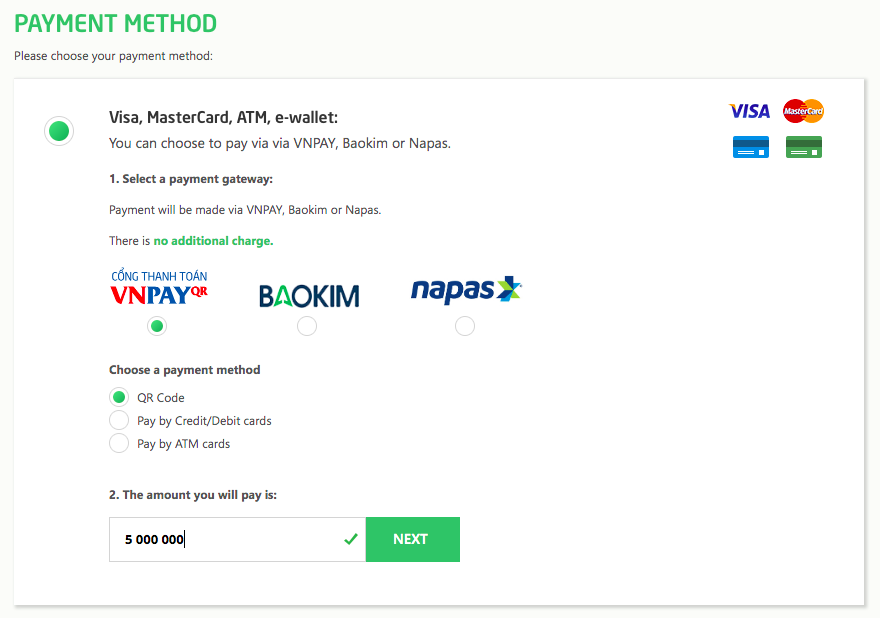The image depicts a payment method selection interface on a website or application with a white background. 

At the top, there is green text in all capital letters that reads "PAYMENT METHOD." Below it, in black text, it says, "Choose your payment method."

In a centrally located white box:
- On the left side, there is a green circle. Accompanying this circle is black text listing "Visa, MasterCard, ATM, eWallet."
- On the right side, there are logos for Visa, MasterCard, and Global, presented in blue, red, and orange respectively.

Below the MasterCard information, it states in black text that users can choose to pay via "VNPAY, BACMO, or NAPIS," which appear to be payment options not commonly used in the United States. It further elaborates, stating, "Once selected payment gateway, payment will be made via VNPAY, BACMO, or NAPIS." Following this, in green text, it mentions that there is "No Additional Charge."

Logos for VNPAY, BACMO, and NAPIS are shown in red and blue, red and green, and blue respectively, with NAPMO being the selected option.

Additionally:
- There is black text that reads "Choose payment method."
- Beside this text are white circles, some with a green fill indicating selection options: "QR code," "Pay by Credit/Debit Card," or "Pay by ATM."

At the bottom of the box:
- There is an indication of the amount to be paid, written as "5 million" separated with spaces for clarity: "5 000 000."

Adjacent to the payment details, a toolbar is visible with a green check mark and a green box containing the white text "Next."